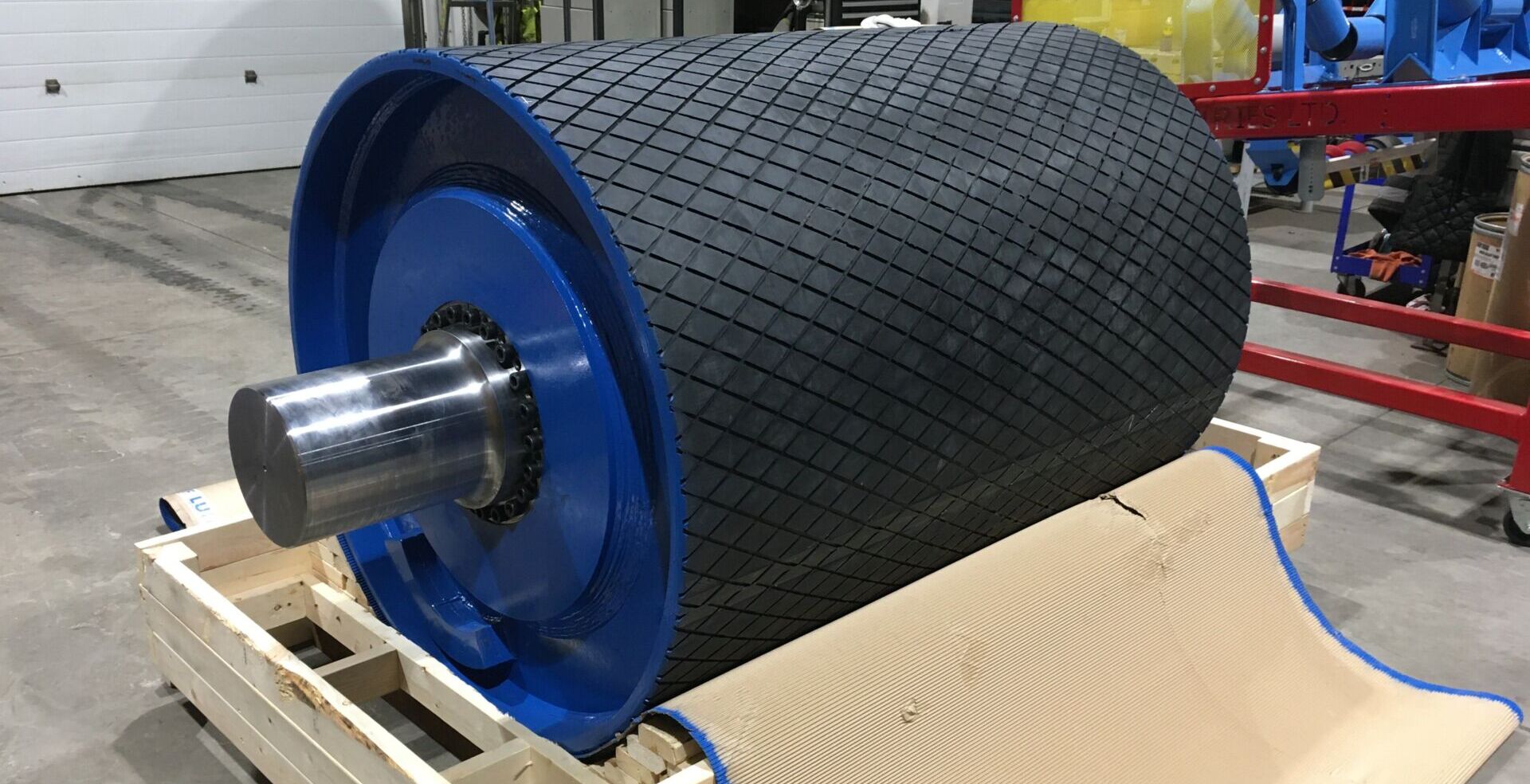The image depicts an indoor manufacturing setting centered around a large cylindrical object that appears to be an industrial roller. This roller rests on a light-colored, unfinished wooden pallet situated on a concrete floor. The body of the roller is coated with a black rubber padding featuring a diamond-crossed tread design, while its circular end is a vibrant metallic blue. Protruding from the center of the cylinder's blue end is a massive silver metal rod. To the right of the image, a red shelving unit holds various blue and yellow items. An overhead garage door is visible in the background, indicating an industrial or warehouse environment. The scene is well-lit, showcasing the details of the device and surroundings, and there is no text present in the image.